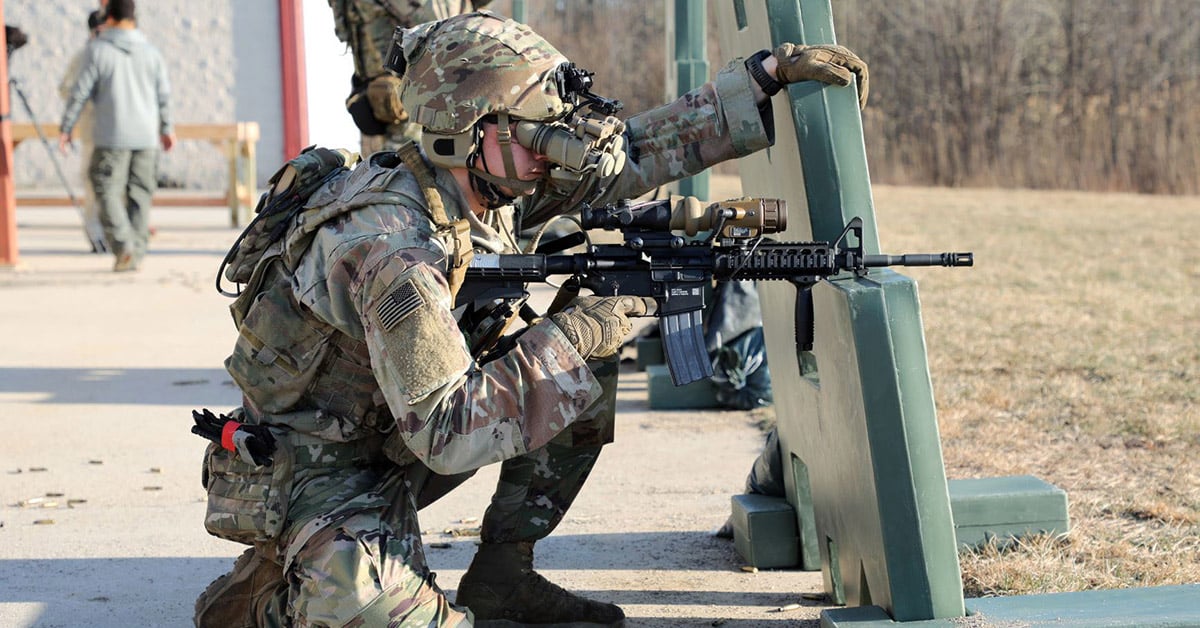The image depicts an American soldier in a kneeling position on one knee, heavily equipped with various army gear. He is dressed in camouflage fatigues in shades of green and brown, with a small backpack and multiple gear strapped to his outfit. An American flag is visible on his arm. On his camouflaged helmet, there are high-tech binoculars or rangefinders, possibly advanced thermal or ultraviolet optics. The soldier grips a black, modern M-16-style rifle, which is equipped with a scope that he is not currently using. Instead, he uses the binoculars while resting his arm on a dark green plastic barricade. The stock of his rifle rests on this same barrier. He is wearing gloves and a black watch. In the background, several other individuals are visible, some in uniform and some not, suggesting that this scene takes place at a shooting range or in an army training scenario.